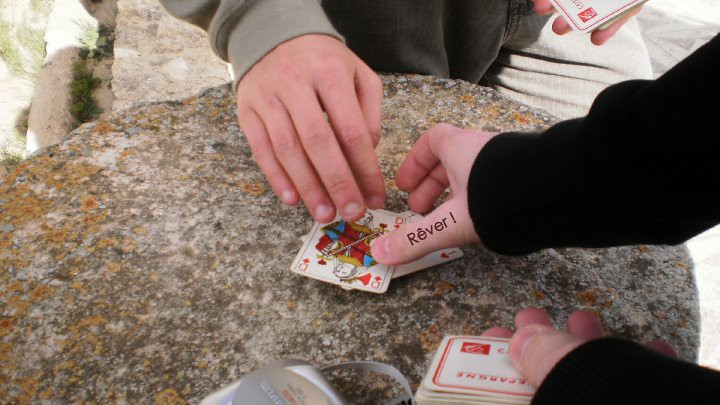Two individuals are engaged in a game of cards atop a large, dark gray rock speckled with patches of yellowish-brown lichen. The scene is bathed in natural light, possibly sunlight filtering from the back left corner where the rocks appear lighter. At the top of the image, a white male with a long-sleeved light green or gray jacket is reaching towards the playing cards without touching them. His other hand, visible in the top right corner, is holding a few face-down cards with white backs bordered in red, adorned with some red text. 

In contrast, another white male's hands, wearing a long-sleeved black sweatshirt, are seen from the right of the image. His right hand is on the cards, and the thumb bears black text reading "R-E-V-E-R!"—the nature of which is unclear whether it's a tattoo or an overlay in the image. His left hand also holds additional face-down cards similar in design. 

On the rock's face, a red Queen of Diamonds and a red Seven of Hearts are visible, though the latter is slightly obscured. A rectangular gray item with a matching gray strap rests at the bottom center, hinting at additional gear or personal effects brought by the players. 

The image captures a serene yet intriguing moment of outdoor leisure, set against the textured backdrop of nature's own game table.